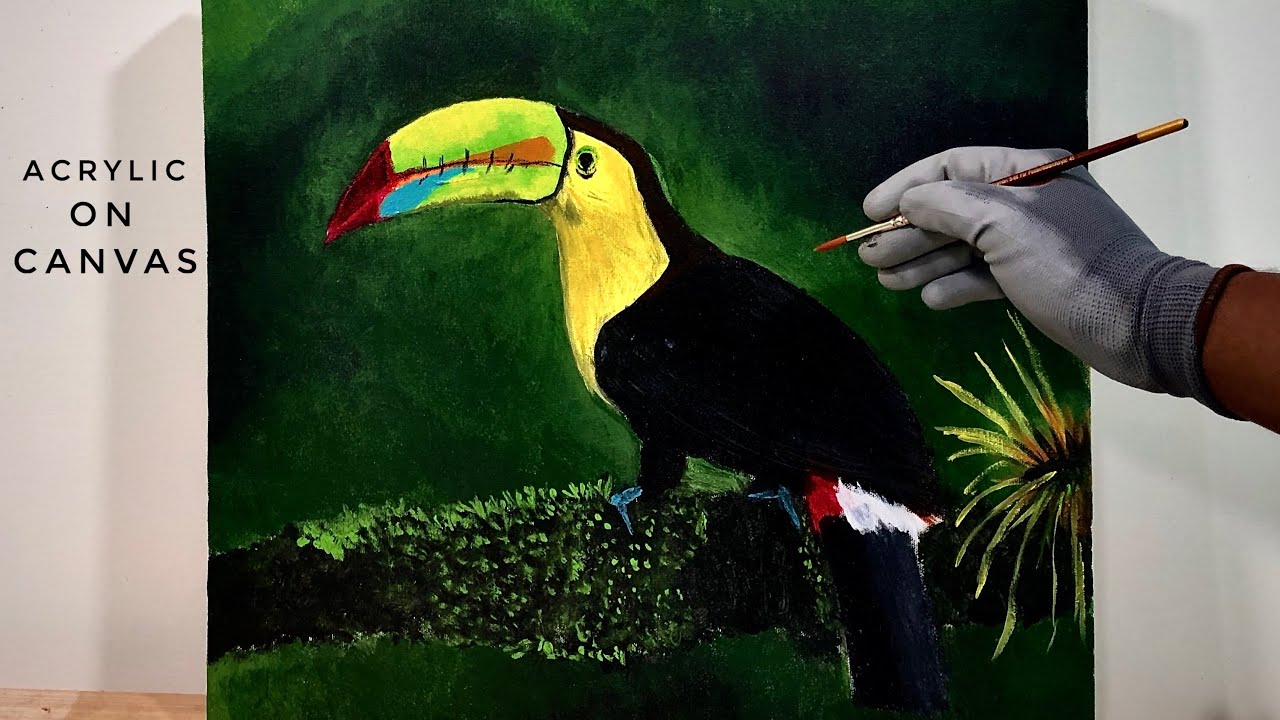A detailed image portrays a vibrant painting process. Framed by a gray border, the scene is wider than it is tall. On the left side, the text "acrylic on canvas" identifies the medium. On the right, a hand donned with a gray glove skillfully wields a paintbrush over a canvas with a rich green background. The painting in progress features a striking toucan perched on a thick, black branch adorned with green foliage. The toucan's body is predominantly black, accented with red and white tail feathers, a bright yellow neck and face, and a beak that showcases a spectrum of colors—green, yellow, orange, blue, red, and purplish hues. A small plant or flower is visible on the lower right side of the canvas beneath the artist's hand. The meticulous details of the foliage and the bird's textured feathers lend a three-dimensional quality to the artwork, capturing the viewer's attention with its vivid realism.